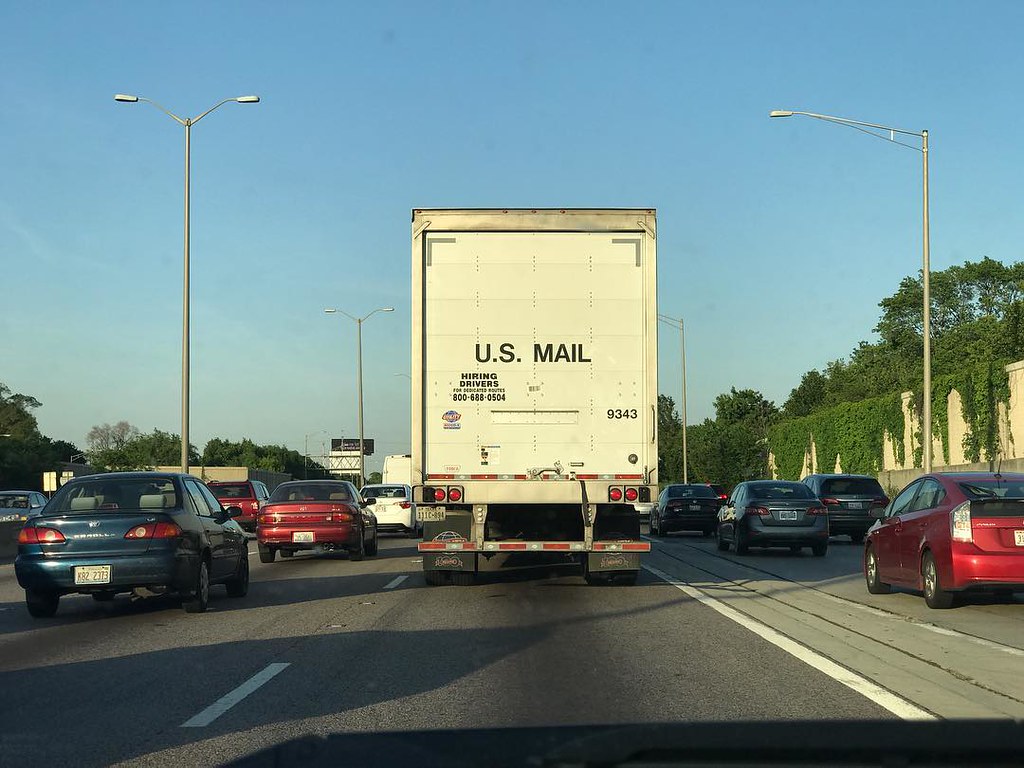A photograph captured from within a vehicle on a busy American freeway showcases a clear, open blue sky above and multiple lanes filled with cars. Dominating the center lane of this expansive, six-lane highway is a large white truck bearing the US Mail logo. This truck prominently advertises hiring drivers, with a phone number displayed on the lower left side of its rear door. Surrounding the truck are various vehicles in hues of blue, red, silver, and white, including Toyota Corollas, a white van, and a Toyota Prius. To the right of the freeway, a vibrant green ivy cascades down a white stone barrier wall, while trees are visible beyond. Streetlights and distant street signs dot the central reservation, guiding the flow of traffic along the clearly marked white lines on the roadway.